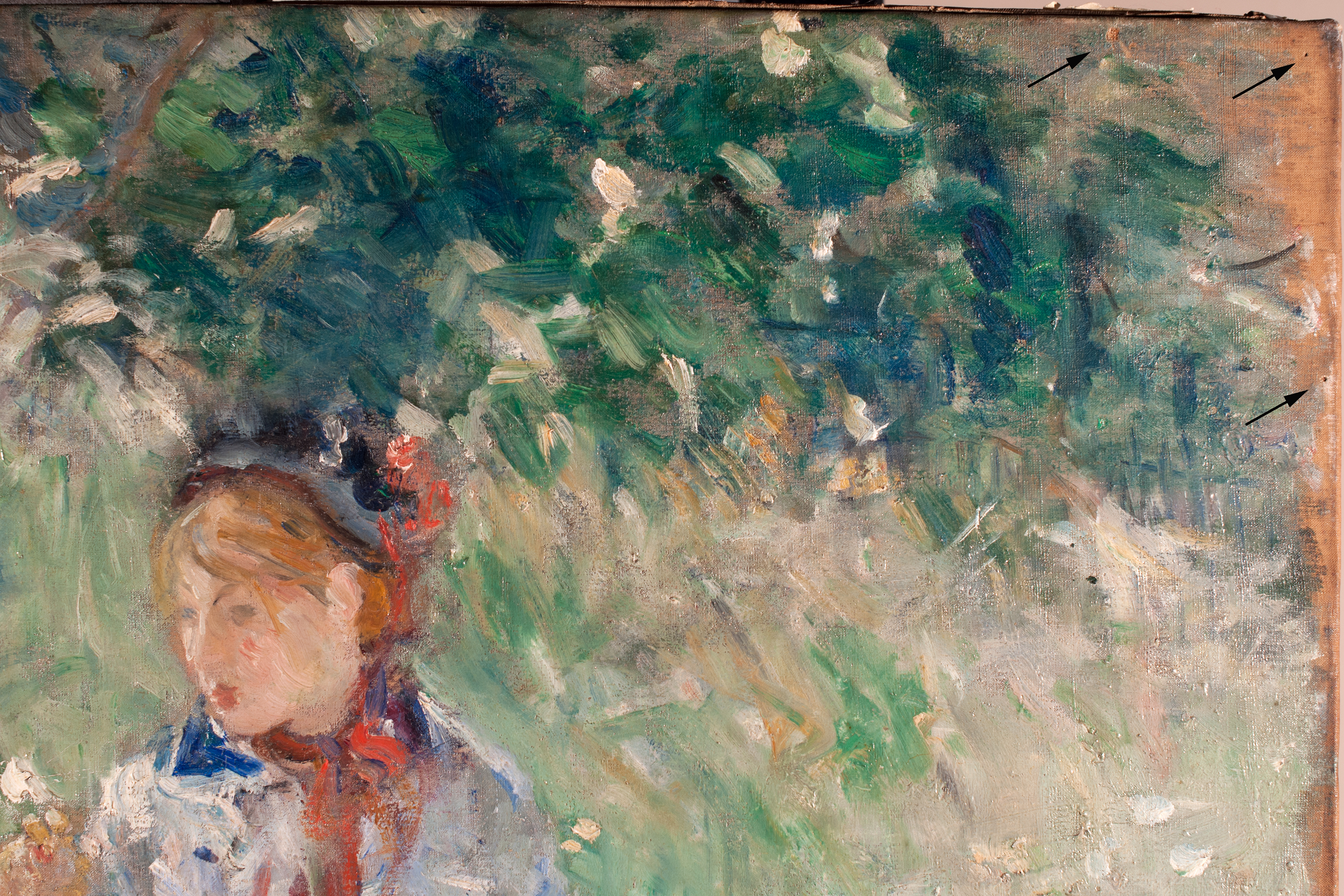This abstract and somewhat blurry painting features a woman positioned in the bottom left corner, visible from her chest up. She has a head turned slightly to the left and down. She has short blonde or reddish-brown hair, bright red lips, and blackish eyes. Adorning her head is a gray hat with black and possibly red ribbons or accents on top. She is dressed in a white shirt with a blue collar and a red handkerchief or scarf around her neck. The bottommost corner of the painting shows hints of flowers in red, yellow, and white hues, perhaps held in her hand or growing nearby. The background consists of a whimsical mix of green, white, and tan streaks, suggestive of a floral or greenery setting but not overly defined. About halfway up, the background transitions to gray shading. In the top right corner, three thin black arrows point diagonally upwards and to the right, drawing attention to the painting's edge. The overall style evokes a sense of whimsy and abstraction, with colors and shapes blending to create a partially defined scene.